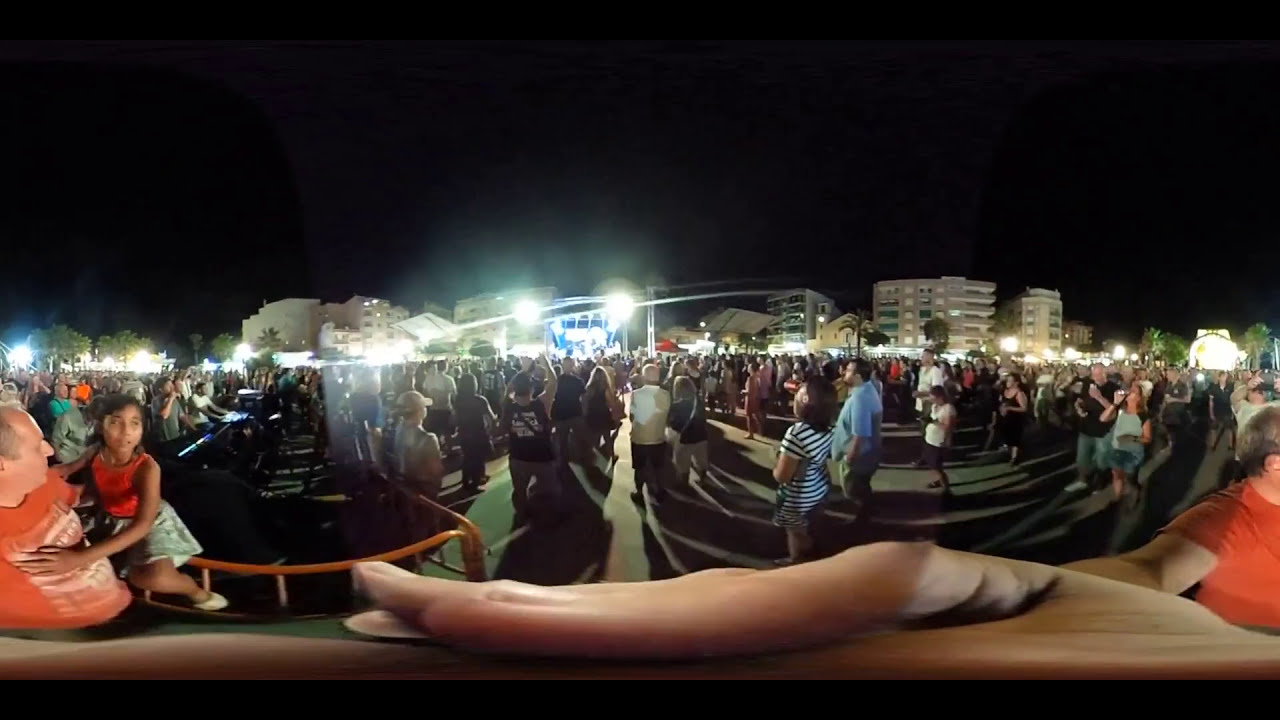The photographic image captures a bustling nighttime city street scene during what appears to be an outdoor festival or concert, from the viewpoint of the person taking the picture. The wide-angle lens exaggerates the appearance of the photographer's thumb in the foreground. The setting is defined by tall, white, multi-story apartment buildings and green trees that frame the scene. The black sky highlights the well-lit plaza where the crowd has gathered.

In the lower left-hand corner, a white man in an orange t-shirt is holding a Hispanic girl, around 5 or 6 years old, wearing an orange tank top and a blue skirt, both looking upwards. The mid-ground is filled with numerous people whose backs are mostly turned towards the camera, facing what seems to be a distant stage. Prominent among them are a woman in a black and white striped shirt, a man in a blue shirt, and several other individuals, emphasizing their upward gaze.

The festival ambiance is further accentuated by the bright lights illuminating the scene, despite the dark night sky. The entire crowd is standing on a blacktop in the plaza, with a mix of different colored clothing visible among them, contributing to the vibrant, lively atmosphere of the event.